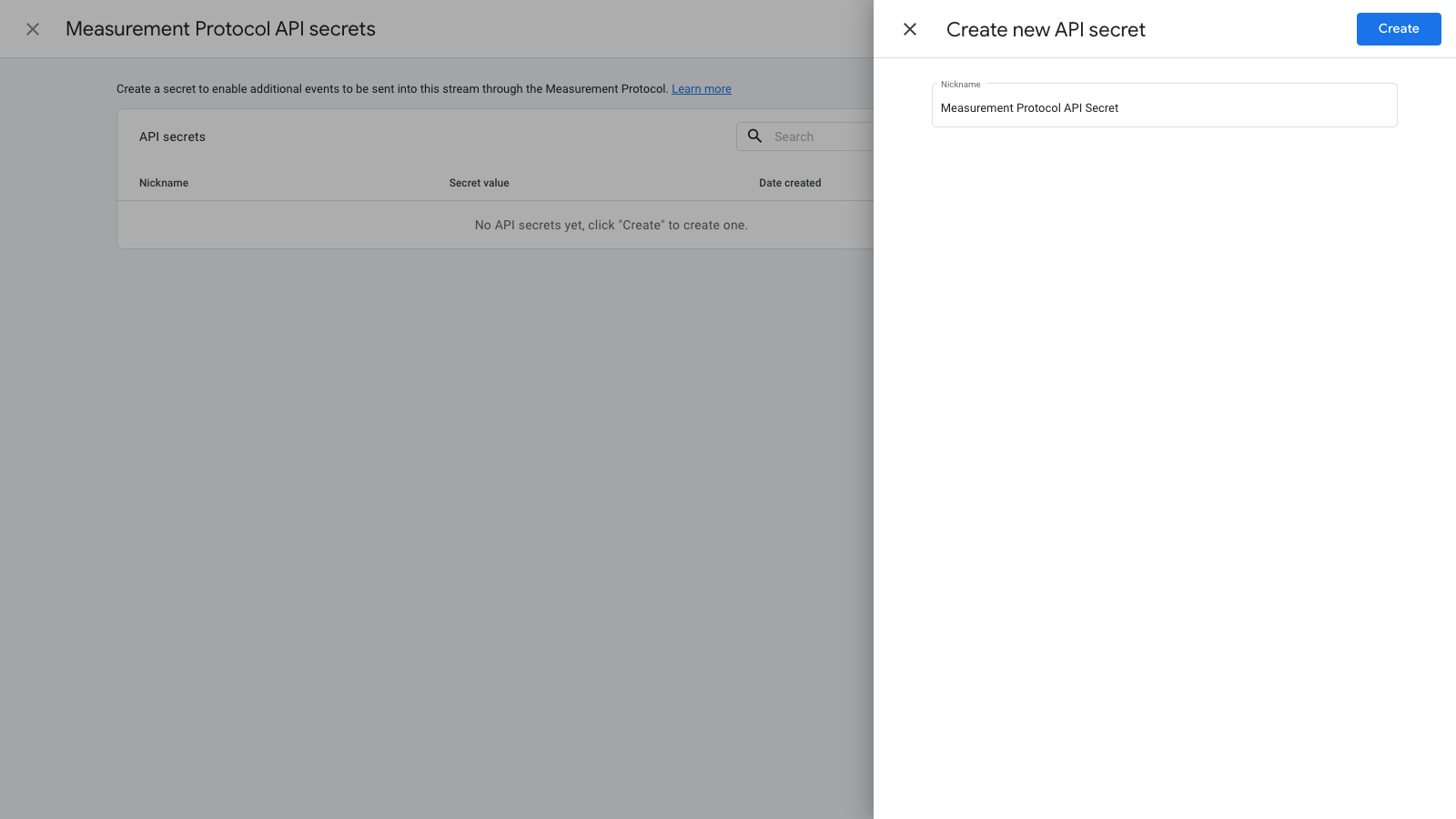The screen is divided into two sections: a gray left side and a white right side. The left side, resembling an overcast gray, features a top bar that reads "Measurement Protocol API Secrets." Below this, the text states, "Create something to enable additional events to be sent into this stream through the measurement protocol," with an underlined "Learn More" link in blue. Underneath, there is a labeled section called "API Secrets," which includes a search bar at the top right under the labels "Nickname," "Secret Value," and "Date Ordered." Just below this is a message indicating that there are currently no API secrets, stating, "No API Secret Yet. Click Create to create one."

On the white right side of the screen, a gray "X" is positioned at the top, next to the text "Create New API Secret." In the far top right corner, a prominent blue button labeled "Create" is displayed. A faint line separates this section from the bottom, where there is another search bar labeled "Measurement Protocol API Secret."